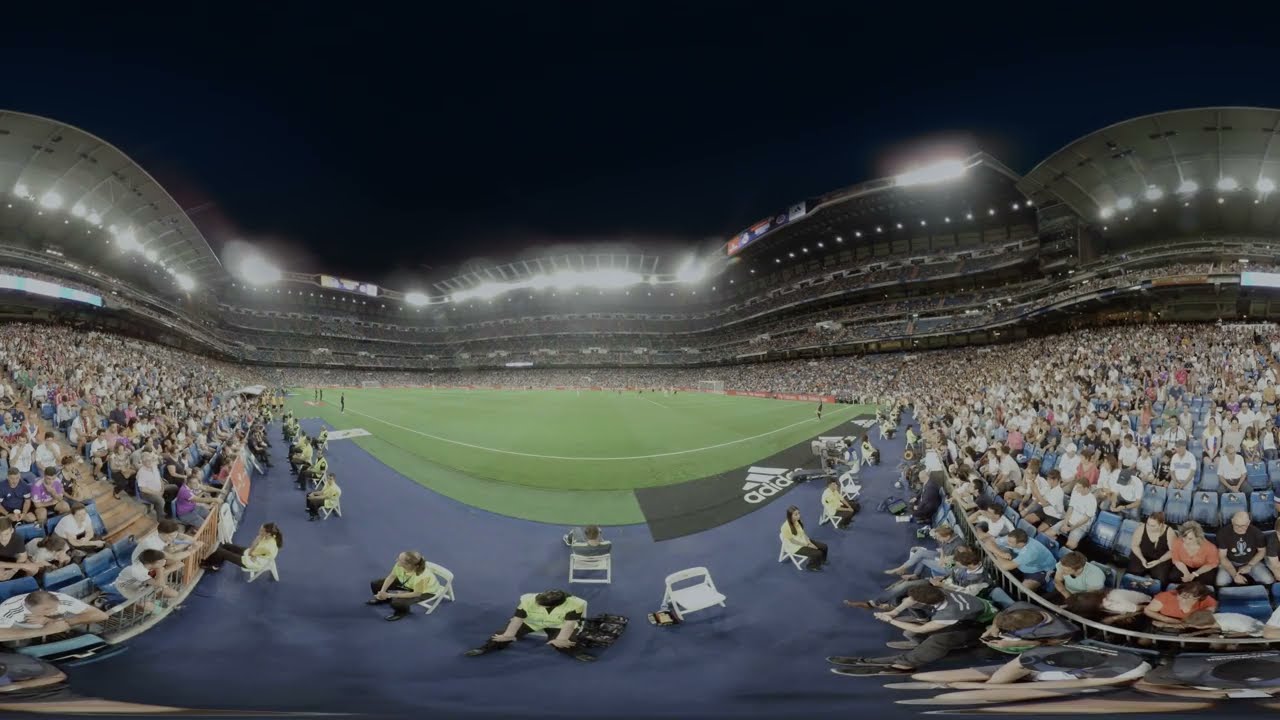This panoramic image showcases the iconic Real Madrid soccer stadium in a uniquely divided, two-scene composition. The lower half prominently features a meticulously maintained green field with white lines, which is empty of players. The field takes center stage, bordered by tiers of blue-themed seating that stretch three levels high, with Real Madrid CF written in bold white letters along the bottom seats. Above these, an upper concourse with multiple windows spans the breadth of the stadium, topped by a sophisticated lighting system adorned with advertisements and banners showcasing logos, possibly including Adidas. The sky overhead is a clear blue-gray, adding to the open, airy feel of the open-ceiling stadium. The outer sections of the stands appear whitish, giving the image a symmetrical and balanced look. The right side of the image intriguingly features a swirling green landscape, enhancing the visual appeal and depth of the photograph.